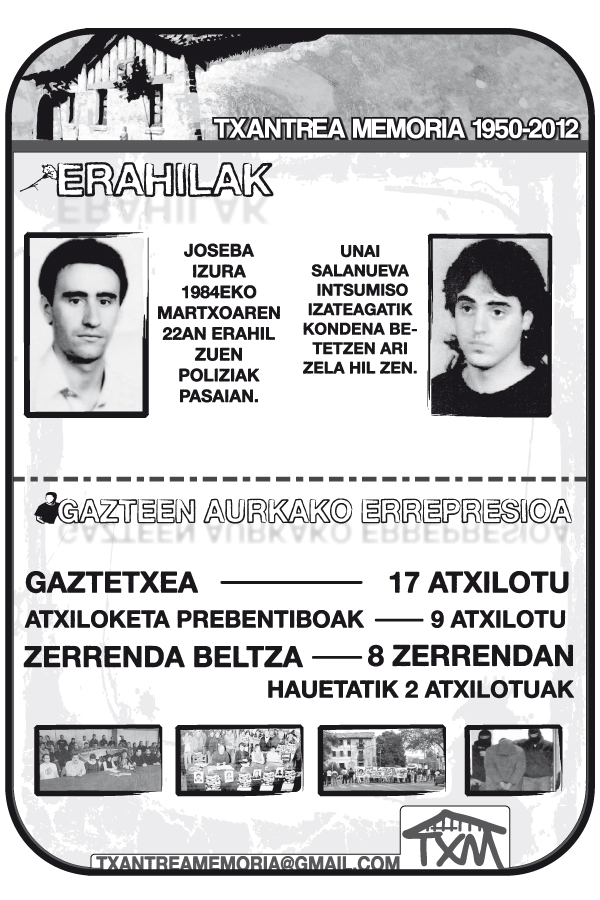The black-and-white poster, written in an unknown language, is rectangular and vertical, featuring a narrow black border. At the top, on the left, there's a photograph of a house with white text to the right reading "T-X-A-N-T-R-E-A M-E-M-O-R-I-A, 1950 to 2012." Below this, in white letters outlined in black, it says "E-R-A-H-I-L-A-K." The center of the poster shows two black-and-white portraits: the left portrait depicts a man with dark hair, heavy eyebrows, dark eyes, and fair skin, while the right portrait displays a younger man with shoulder-length feathered black hair, heavy eyebrows, dark eyes, and fair skin, facing slightly to his right. Between these portraits is dark text including "Gaston, Eurico, Euripresso."

Beneath the portraits, there are further dark text lines, followed by four small pictures at the bottom. The pictures portray various scenes: groups of people, a building with individuals standing outside, and two masked men holding another person hostage. In the bottom right corner is a logo with the letters "TXM" beneath a roof-like design, and the text "Texantra Memorial at gmail.com."